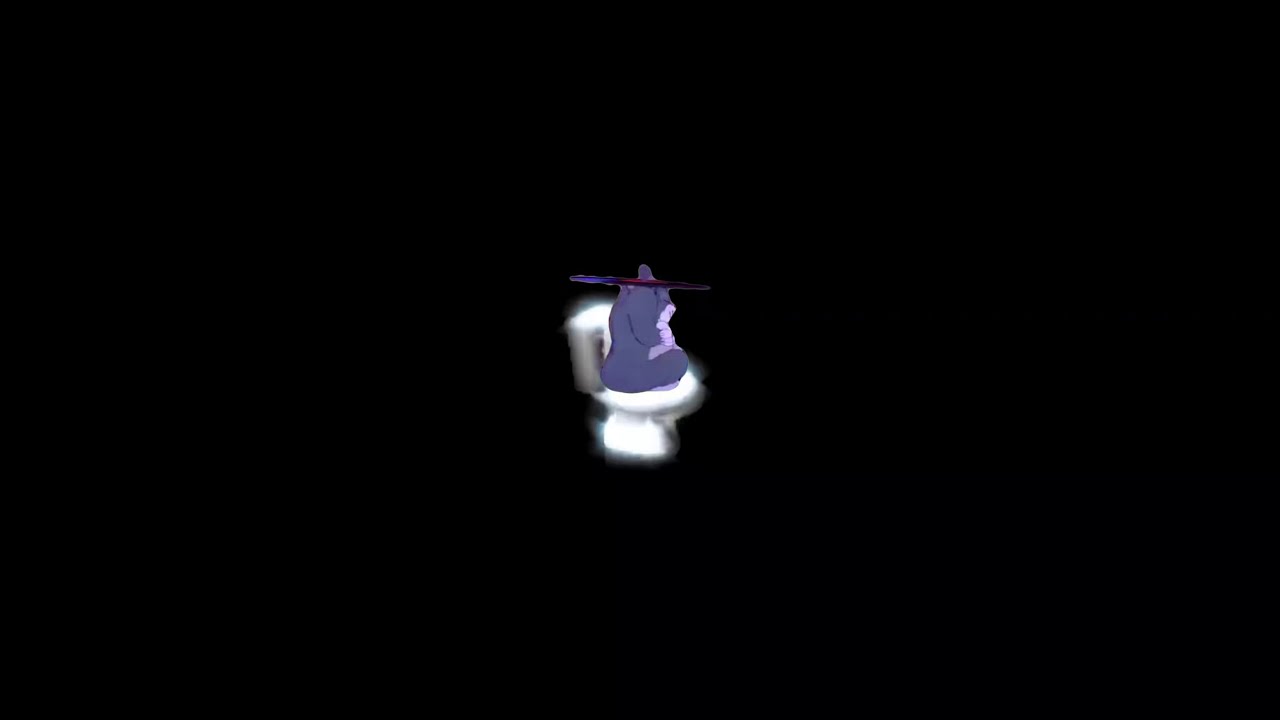In the center of a horizontal rectangular image with a solid black background sits a small, purple cartoon animal on a bright white, realistic toilet. The animal, resembling a pudgy, digitized figure with darker purple fur and a lighter purple chest and underbelly, is facing to the right. It is cross-legged, with its legs tucked upwards onto the toilet seat, obscuring them from view. Its mouth and the tips of its paws are also lighter in color, possibly white, and it has black whiskers. The animal appears to be wearing a small hat that looks like a black and red witch's hat or perhaps a surfboard. The toilet, which faces to the right as well, appears to be glowing slightly due to poor image quality, adding to the contrast between the realistic white toilet and the cartoonish character. The entire image is relatively pixelated and blurry around the edges.